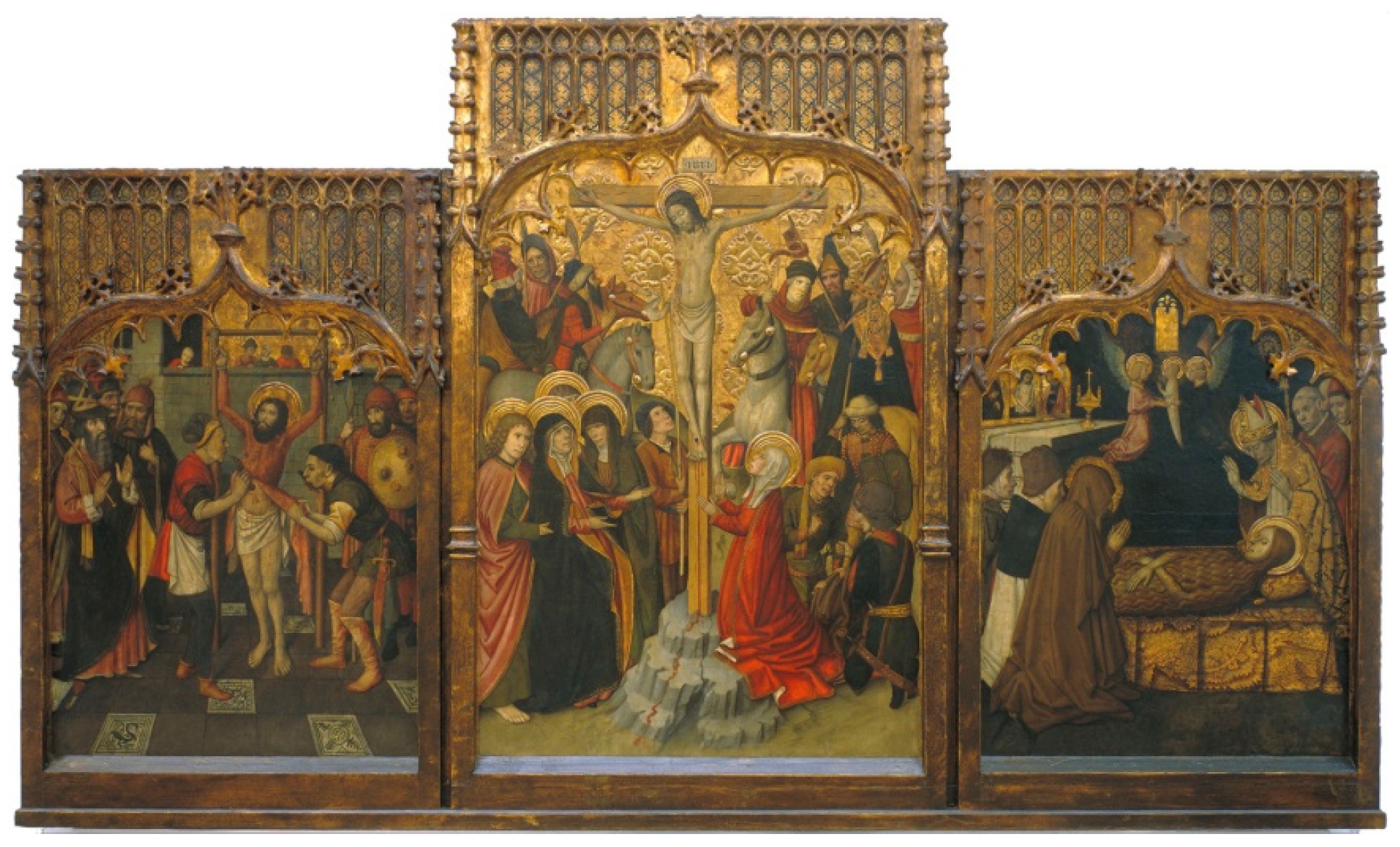This detailed triptych religious artwork, meticulously carved and painted on wood, depicts the final moments and aftermath of Jesus Christ's life. The central and largest panel features Jesus on the cross, surrounded by a grieving Mary Magdalene in a red dress kneeling at his feet, along with several women and soldiers on horseback. The intricately carved wooden frame enhances the gold leaf painting. The left panel portrays Jesus being prepared for crucifixion, with figures removing his clothing and numerous onlookers, including guards. The right panel depicts a solemn funeral scene, with Jesus laid to rest and mourners praying around him. Traditional Catholic golden halos adorn the heads of the holy figures, emphasizing their sanctity and importance. The lower parts of the frames are simpler, but the tops are elaborately carved, showcasing extraordinary woodwork and adding to the piece's overall grandeur.